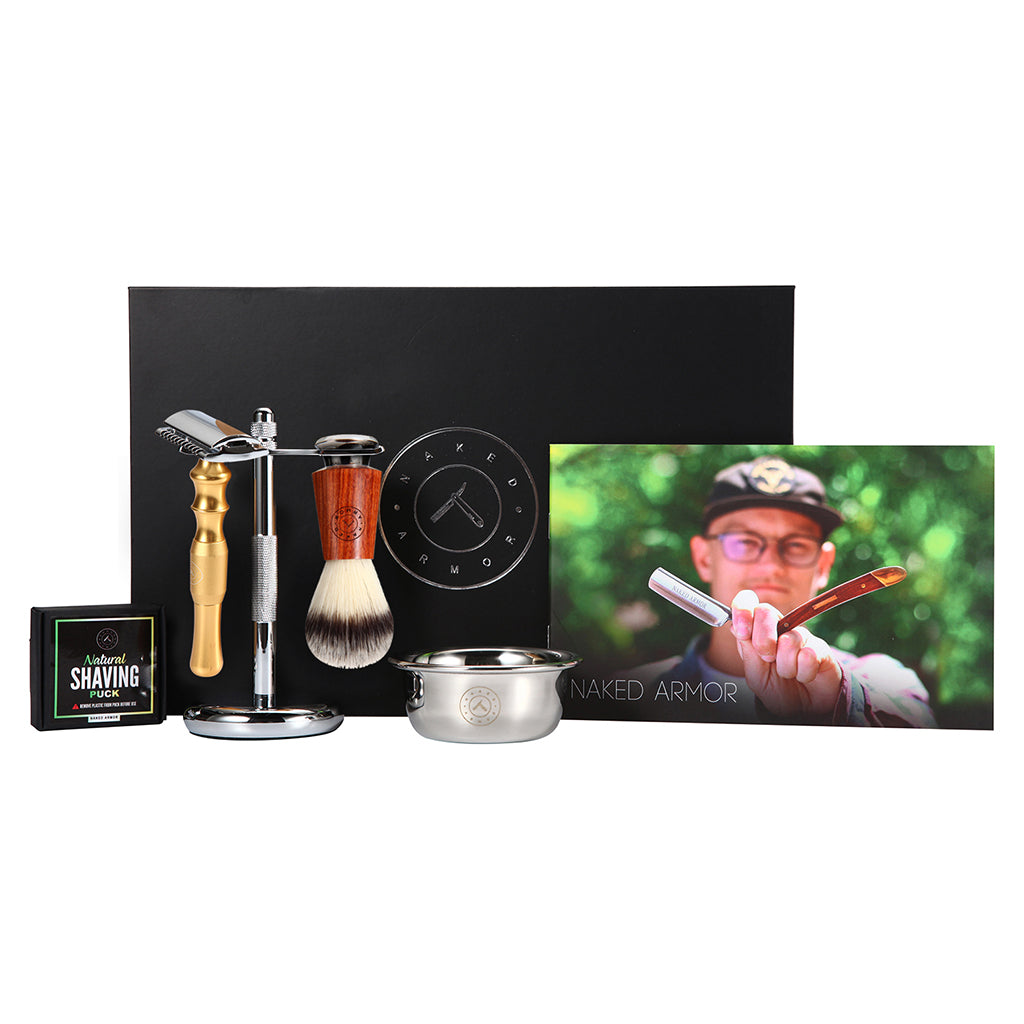This advertisement photograph showcases a premium straight razor shaving set known as Naked Armor. The focal point of the image is the elegantly designed shaving equipment, prominently featuring a razor, a small lather bin for shaving cream, and a shaving brush, all suspended on a sleek silver metal stand. The shaving cream bowl is also crafted from silver metal, exuding a sophisticated aesthetic. To the left, you notice a box labeled "Natural Shaving Puck" in black with green trim. 

The right side of the composition reveals a young man extending a folding straight razor towards the camera, emphasizing the dual elements of blade and wooden sheath. The man, wearing glasses and a black hat, stands against a green background, adding a modern, relatable touch to the advertisement. In the background of the shaving set center, another black box features the intricate Naked Armor logo—a circular emblem with a V-shaped straight razor.

Together, the multifaceted image combines photorealistic and illustrative elements, providing a detailed and comprehensive view of the sophisticated Naked Armor shaving set.